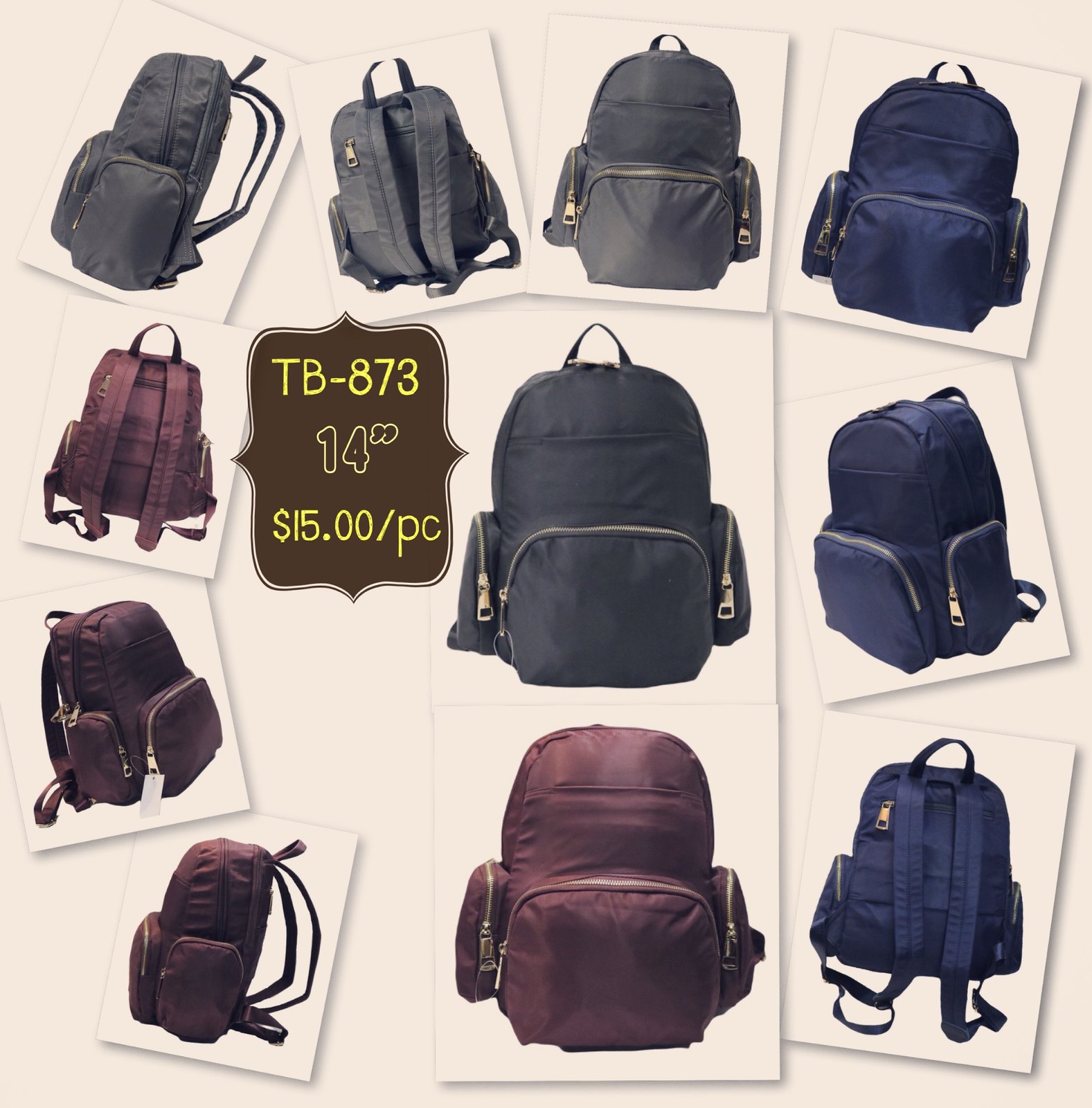The image is a detailed, collage-style advertisement for backpacks, likely sourced from a wholesale website such as AliExpress or Alibaba. The background is plain white with a sepia filter applied, giving it a vintage look. The collage showcases 11 backpacks in total, all of the same design but available in three different colors: black, maroon (burgundy), and navy blue.

Each backpack is featured in multiple angles, allowing viewers to see various details such as the zippered front pocket, side pockets, and adjustable straps. The layout of the images is organized into three rows. The top row includes three black backpacks and one blue backpack. The middle row contains images of one backpack in each color—black, maroon, and navy—surrounding a central brown rectangular box. This box features yellow text displaying the product number TB-873, dimensions of 14 inches, and a price of $15 per piece. The bottom row presents three maroon backpacks and one navy blue backpack.

Despite some inconsistencies in the pricing labels, with one area noting $14.99 and another $15, the main focus remains on the visual representation of the backpacks' features and color options. Overall, this image effectively serves as a comprehensive advertisement for potential buyers interested in wholesale backpack purchases.